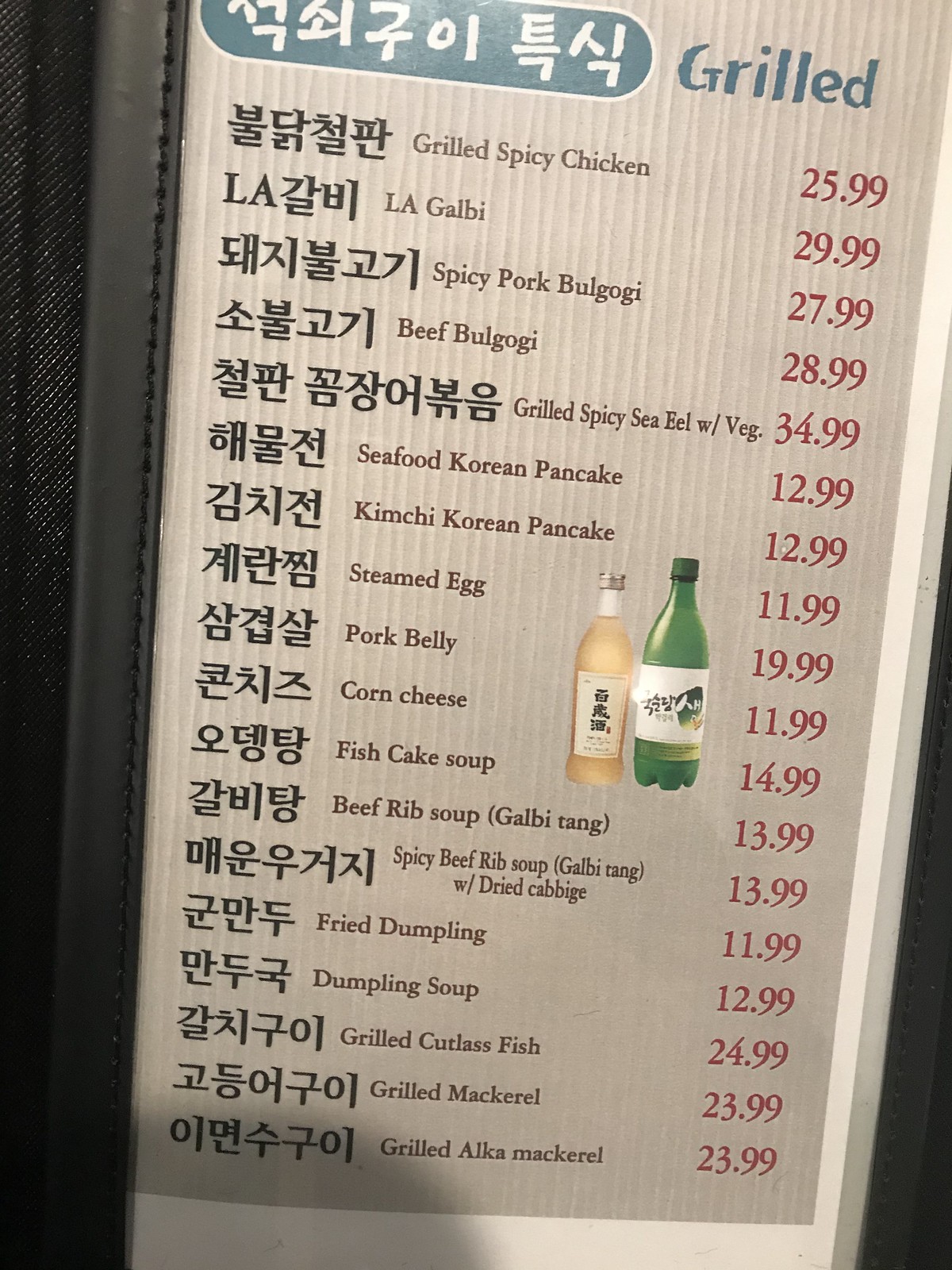The image appears to be a bilingual menu from a restaurant, featuring both an Asian language (potentially Korean, Japanese, or Chinese) and English. The menu is displayed on a blue background with white text. The categories of food and beverages include grilled items, soups, pancakes, and traditional Korean dishes. Here is a detailed breakdown of the menu items along with their prices:

- Spicy Grilled Spicy Chicken: $25.99
- LA Galbi: $29.99
- Spicy Pork Bulgogi: $27.99
- Beef Bulgogi: $28.99
- Grilled Spicy Sea Eel with Vegetables: $34.99
- Seafood Korean Pancake: $12.99
- Kimchi Korean Pancake: $12.99
- Steamed Egg: $11.99
- Pork Belly: $19.99
- Corn Cheese: $11.99
- Fish Cake Soup: $14.99
- Beef Rib Soup (Galbi Tang): $13.99
- Spicy Beef Rib Soup (Galbi Tang) with Dried Cabbage: $13.99
- Fried Dumpling: $11.99
- Dumpling Soup: $12.99
- Grilled Cutlass Fish: $24.99
- Grilled Mackerel: $23.99
- Grilled Alka Mackerel: $23.99

Additionally, the menu highlights two bottles of Asian alcohol: one in a green bottle and the other in a yellow bottle, which suggests the availability of soju or a similar type of alcoholic beverage.

Overall, the menu provides a comprehensive selection of grilled meats, seafood, traditional Korean soups, savory pancakes, and other popular dishes, catering to various tastes and preferences.